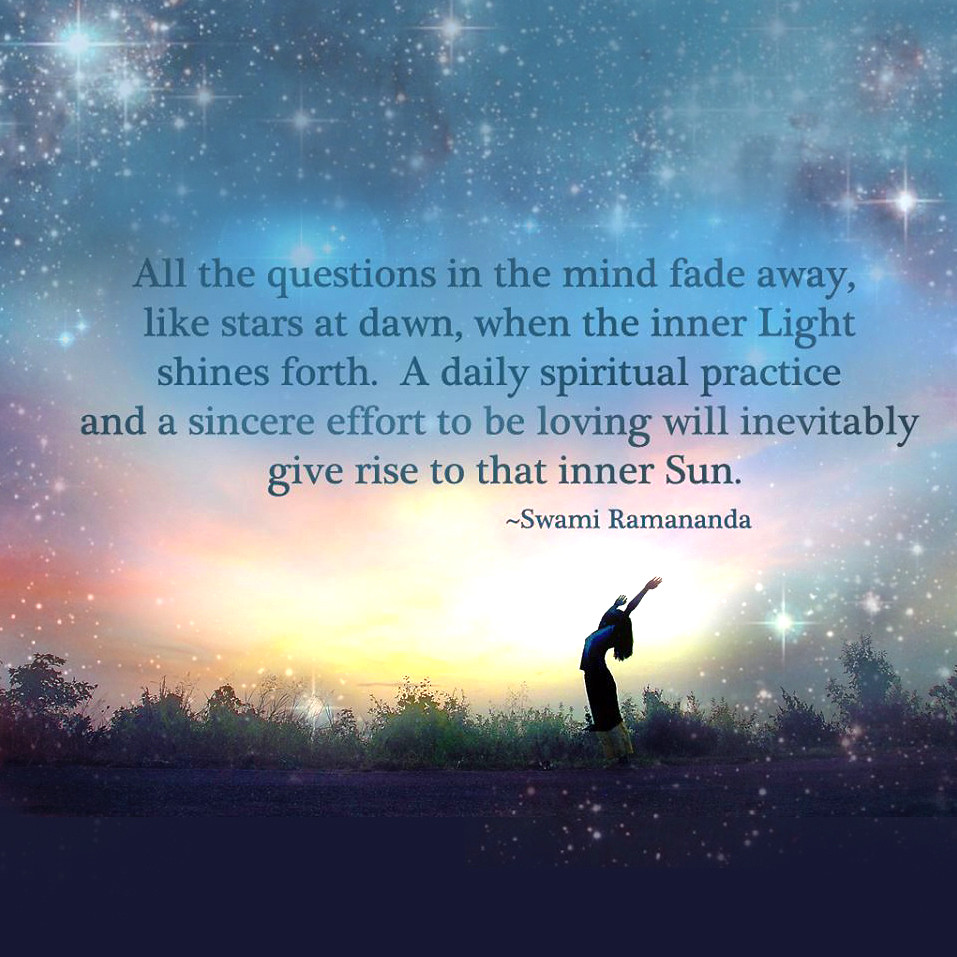In this detailed and vivid illustration, a woman stands in a field at the side of a road, her silhouette dark and indistinct, with arms stretched upwards in a victorious pose. Behind her, lush tall grass nearly mirrors her height, blending into the background. The scene is dominated by a surreal, dreamlike sky: it begins with a brilliant sunset featuring hues of pink, yellow, and orange near the horizon and transitions upward into a faded galaxy design, replete with both bright and subtle stars. This heavenly backdrop serves as the canvas for an inspirational quote in elegant black text that reads, "All the questions in the mind fade away like stars at dawn when the inner light shines forth. A daily spiritual practice and a sincere effort to be loving will inevitably give rise to that inner sun." This quote is attributed to Swami Ramananda and emphasizes the spiritual transformation symbolized by the serene and mystical sky.